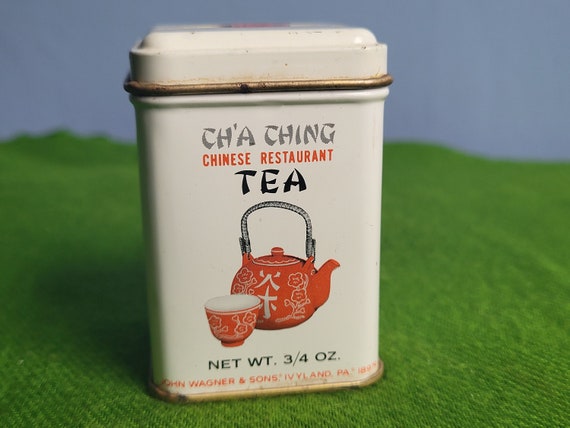The image displays a vintage, rectangular, vertical canister made of metal with an off-white color. The canister has a slightly rusted rim around its lid, which is gold-colored. The front of the canister prominently features the text "Cha Ching Chinese Restaurant Tea" on three separate lines. Below this text, there is an image of a small red teapot with Chinese characters on it and a matching red teacup beside it. The canister also contains detailed text stating "Net Weight 3/4 oz" in black lettering and "John Wagner & Sons, Ivyland, PA" in red lettering. The canister rests on a green cloth that resembles grass, with a medium blue background suggesting the sky. Lighting from the front casts a shadow behind the canister.